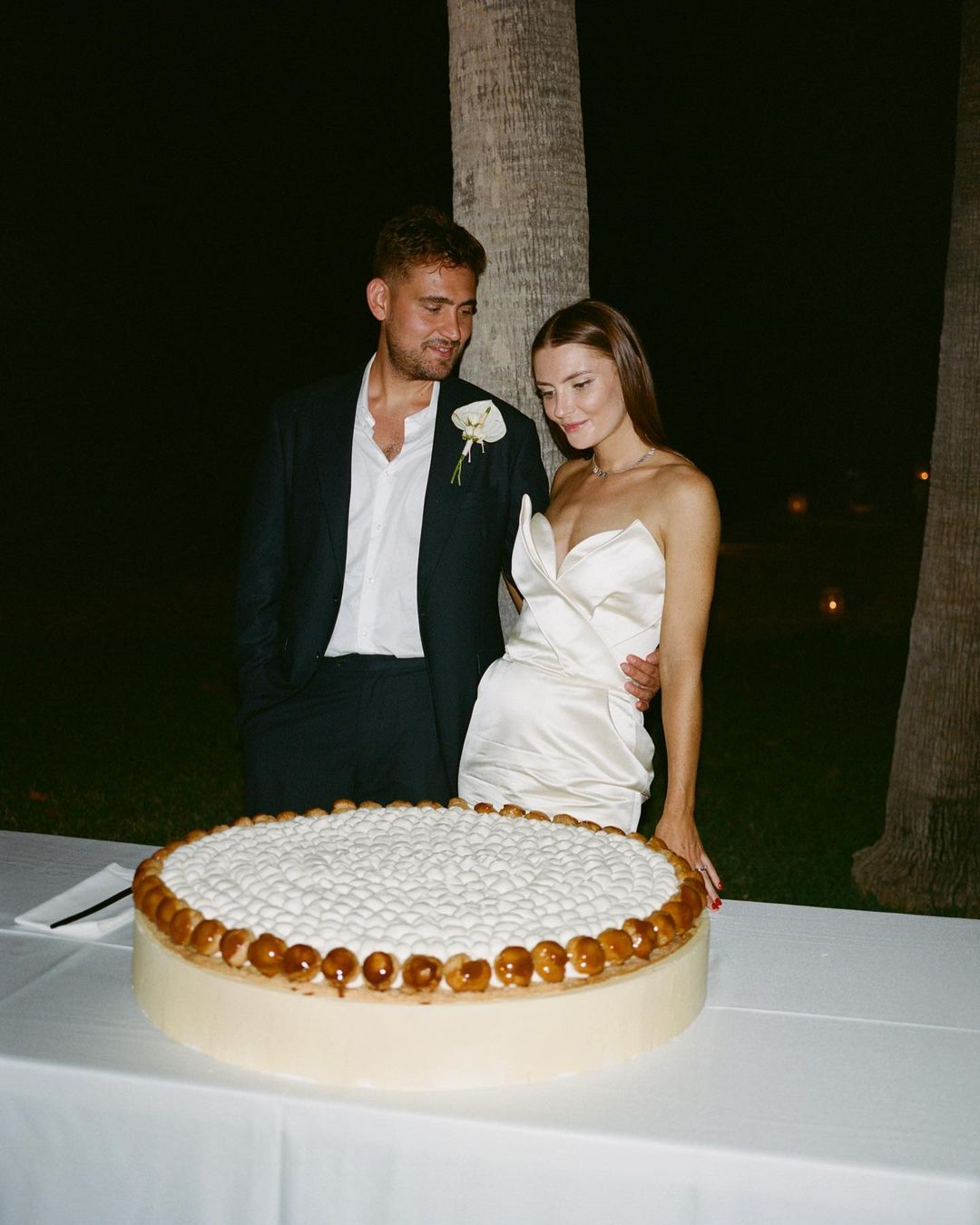In this nighttime wedding photograph, we see a couple standing closely together in front of a long white table, covered with a white cloth, that holds an elaborate cake. The cake is beige, adorned with what appears to be white marshmallows on top, and its circumference is lined with small caramel-coated fruits, such as candied apples. To the left of the cake, a stack of white napkins is topped with a cake knife, ready for use.

The woman is dressed in a sleeveless, flowing white gown, sporting red nail polish on her visible hand that rests on the table. She has brown hair and gazes down at the cake with a look of contemplation or admiration. Beside her stands the man, dressed in a slightly unbuttoned white dress shirt under an open black suit jacket and black pants. He also wears a white flower corsage pinned to his chest and has his arm affectionately wrapped around the woman's waist. He has short dark hair and looks at her lovingly.

Behind them, the backdrop is predominantly black, emphasizing that the event takes place at night, though a couple of trees and some grass can be seen, partially illuminated by the scene's lighting. The overall setting suggests that the photo captures a special moment at a wedding celebration.